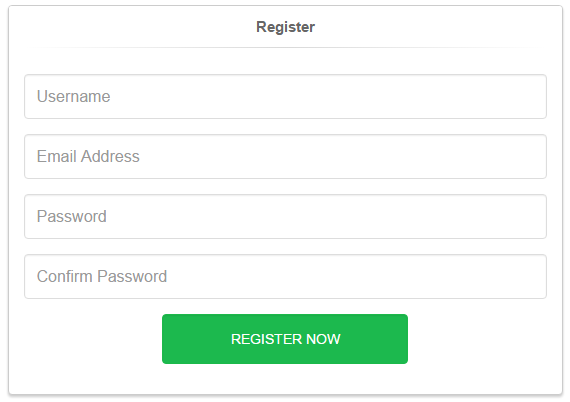The registration pop-up is a horizontally elongated rectangle with a minimalistic design featuring a white background and a very light gray border. At the top, the word "Register" is prominently displayed in black font. Below this, a thin gray line separates the title from the input fields.

There are four input fields, each outlined by a gray line and shaped as long, thin rectangles:
1. The top field is labeled "Username" in gray text.
2. The second field down is labeled "Email Address" in gray text.
3. The third field down is labeled "Password" in gray text.
4. The final field is labeled "Confirm Password" in gray text.

At the bottom of the pop-up, there is a horizontally elongated green rectangle button with "Register Now" written in white text, serving as the registration submission button.

The overall color scheme consists of white, gray, black, and green. The interface is large and clear, ensuring readability even when the image is enlarged.